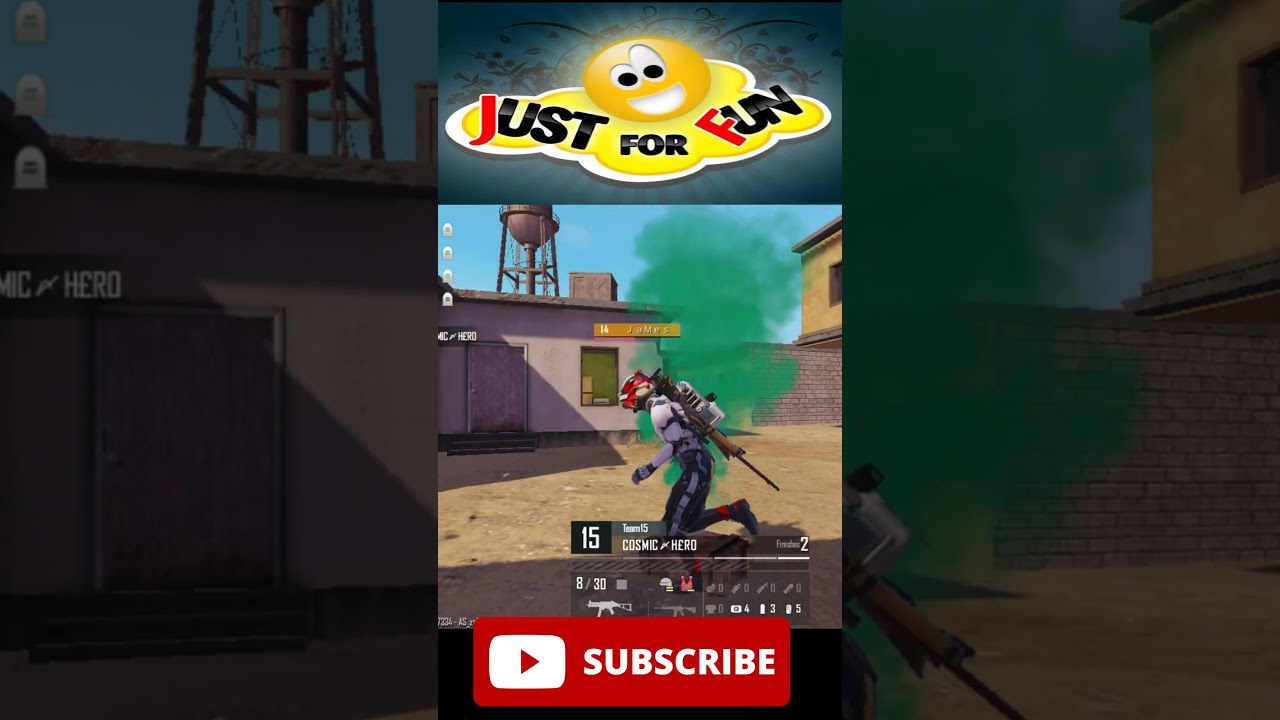This is a detailed screenshot from a video game, featuring an outdoor scene with a dirt courtyard and a flat-roofed building with a water tower in the background. Dominating the center of the image is a fully geared player, James, identifiable by the labeled "14 James" above his head. The player is donned in an outfit resembling motocross racing gear, including a red and white helmet, a white top, black bottoms, long-sleeve jersey, motorcycle gloves, and blue leather pants with white stripes. A rifle is slung behind his shoulder and he seems to have a jetpack or back apparatus attached. The player is enveloped in a green cloud of smoke, possibly denoting action or movement.

Above the player, the top center of the image displays a whimsical yellow cloud with a smiley face emoji and the words "JUST FOR FUN" in a red and black all-caps font, where the letters 'J' and 'F' are red, and the rest are black. Beneath this vibrant headline, information tags read "Team 15 Cosmic Hero" and "8/30". At the bottom of the image, a prominent red text box with the white word "SUBSCRIBE" is situated. The overall composition hints that the game scene may be intended for casual, engaging gameplay, enhanced by the playful top banner and the vibrant details in the character's gear and surroundings.